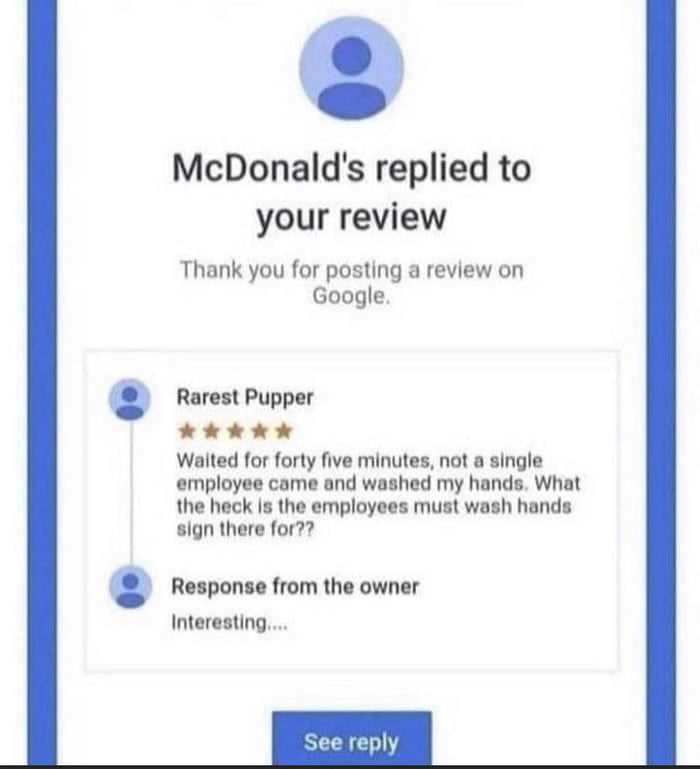This screenshot displays a McDonald's restaurant review and its response on Google. Framed by long blue vertical lines on each side and a thin black horizontal line at the bottom, the image features a blue round profile image placeholder at the top center, with the text "McDonald's replied to your review" just below it. 

The main section of the screenshot includes a rectangular text box containing both the review and the response. The review, authored by Rarest Pupper, grants the restaurant five stars. Despite the high rating, the review humorously reads: "Waited for 45 minutes. Not a single employee came and washed my hands. What the heck is the 'employees must wash hands' sign there for??" 

The owner's response is succinct and slightly enigmatic, simply stating: "Interesting...."